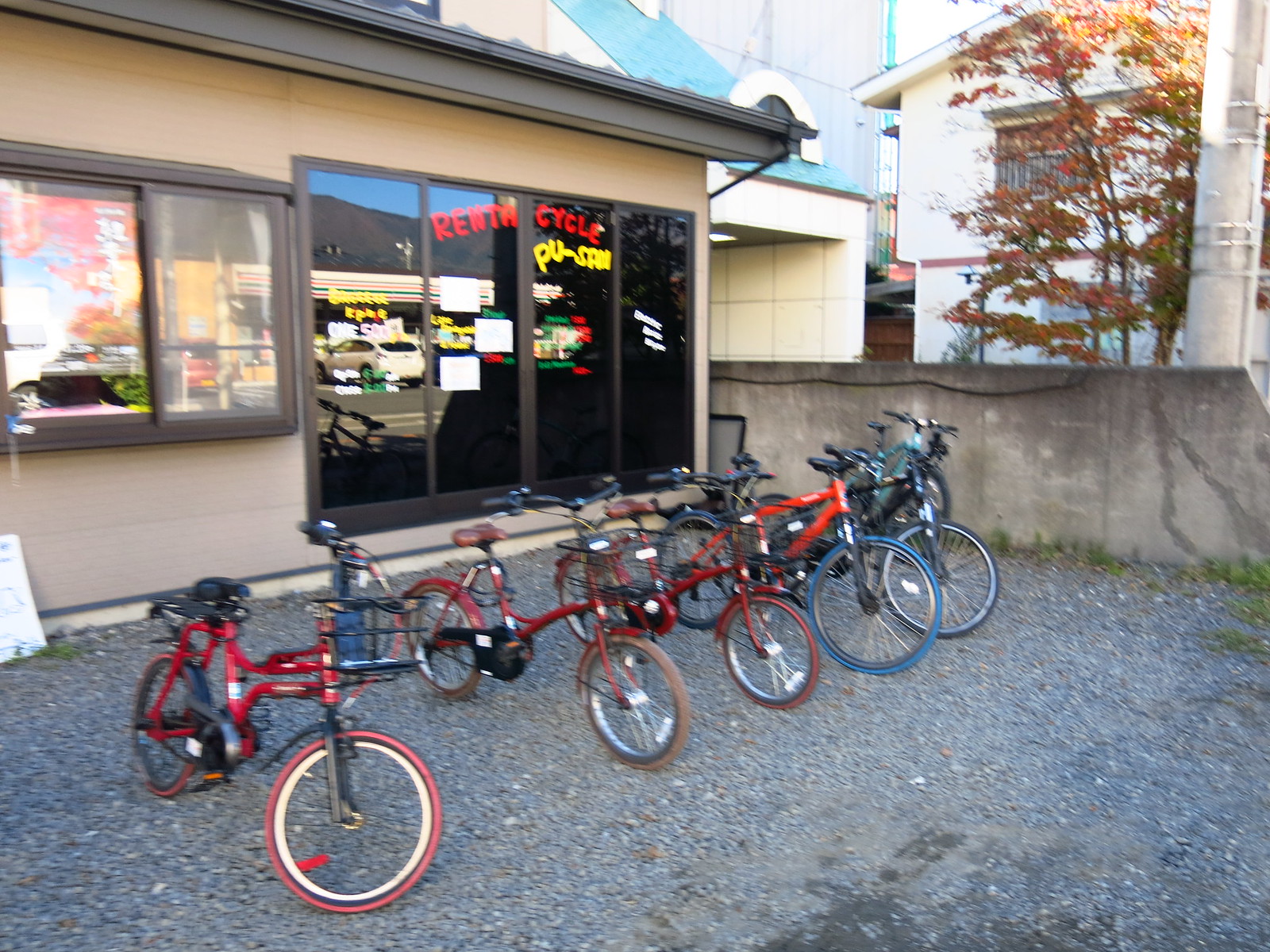In this low-resolution, slightly blurry landscape photograph, we see an exterior scene featuring six bicycles arranged in a row on a blue and grey gravel surface in front of a shop named "Renneth Cycle." The shop itself is characterized by dark, black windows and light brown siding topped by a grey roof truss. A large sliding door prominently displays the shop’s name: "Renneth Cycle" in red letters and "Poussat" in yellow. The scene also includes a series of varied-sized bikes: three smaller-framed red bicycles, followed by an orange bike with blue wheels, and finally a larger bike with a nearly black frame. To the right side of the image, there is a tree with a mix of green and reddish autumn leaves behind a short concrete wall, and further back sits a white house. The ground beneath the bicycles is dotted with grey dirt, lending a rustic backdrop to this small bicycle rental business.